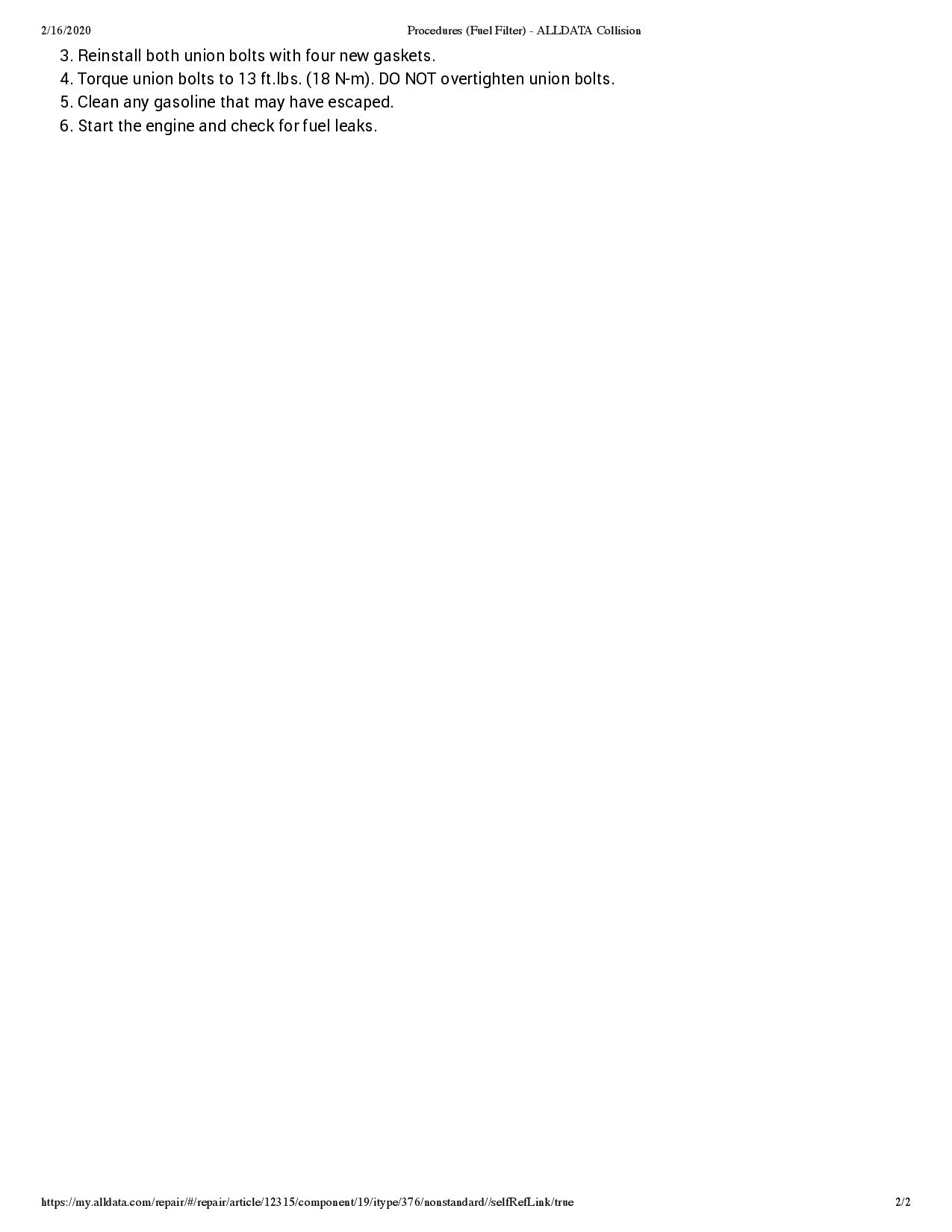In the image, a clear white sheet of paper contains procedural text, with a date of February 16, 2020, prominently displayed in the top left corner. The content consists of detailed steps for a specific maintenance task involving a fuel filter, organized as follows:

1. **Reinstall both union bolts.**
2. **Install new gaskets.**
3. **Torque union bolts to 13 feet-pounds (18 Newton meters).**
4. **Caution:** Do not over-tighten union bolts.
5. **Clean any gasoline that may have escaped.**
6. **Start the engine and check for fuel leaks.**

The bottom of the sheet includes a URL for further information: [myoldata.com/repair/article/123154/components](https://myoldata.com/repair/article/123154/components). This link presumably offers additional context or supplementary details related to the procedures described.